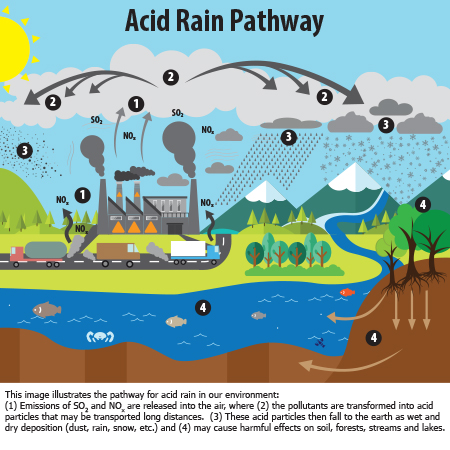This image is an educational infographic that illustrates the pathway of acid rain in our environment. The top of the image prominently displays the title "Acid Rain Pathway" in black text. The sky is a clear blue, providing a vivid background for the various elements depicted in a cartoonish style. 

Central to the infographic is a series of gray arrows indicating both the sources and effects of acid rain. The image features gray clouds emitting sulfur dioxide (SO2) and nitrogen dioxide (NO2), pollutants that transform into acid particles and travel long distances through the atmosphere. The pollutants eventually descend as acid rain, impacting various natural and human-made features illustrated below.

On the left side of the image, there's a bright yellow sun partially covered by gray clouds, some of which are releasing snow. At the base of the mountains, a river flows through a green and white landscape, flanked by lush greenery and brown soil. There is a notable grassland with multiple trees, indicating the terrestrial effects of acid rain. Vehicles drive along a road near a gray factory, emphasizing industrial contributions to the pollution.

The bottom section of the image contains a detailed paragraph in black print, explaining the acid rain process with numbered points corresponding to different parts of the infographic. This highlights the harmful environmental impacts, such as soil degradation and water body acidification. Overall, the visual and textual elements combine to provide a comprehensive overview of how acid rain forms and affects various parts of the ecosystem.